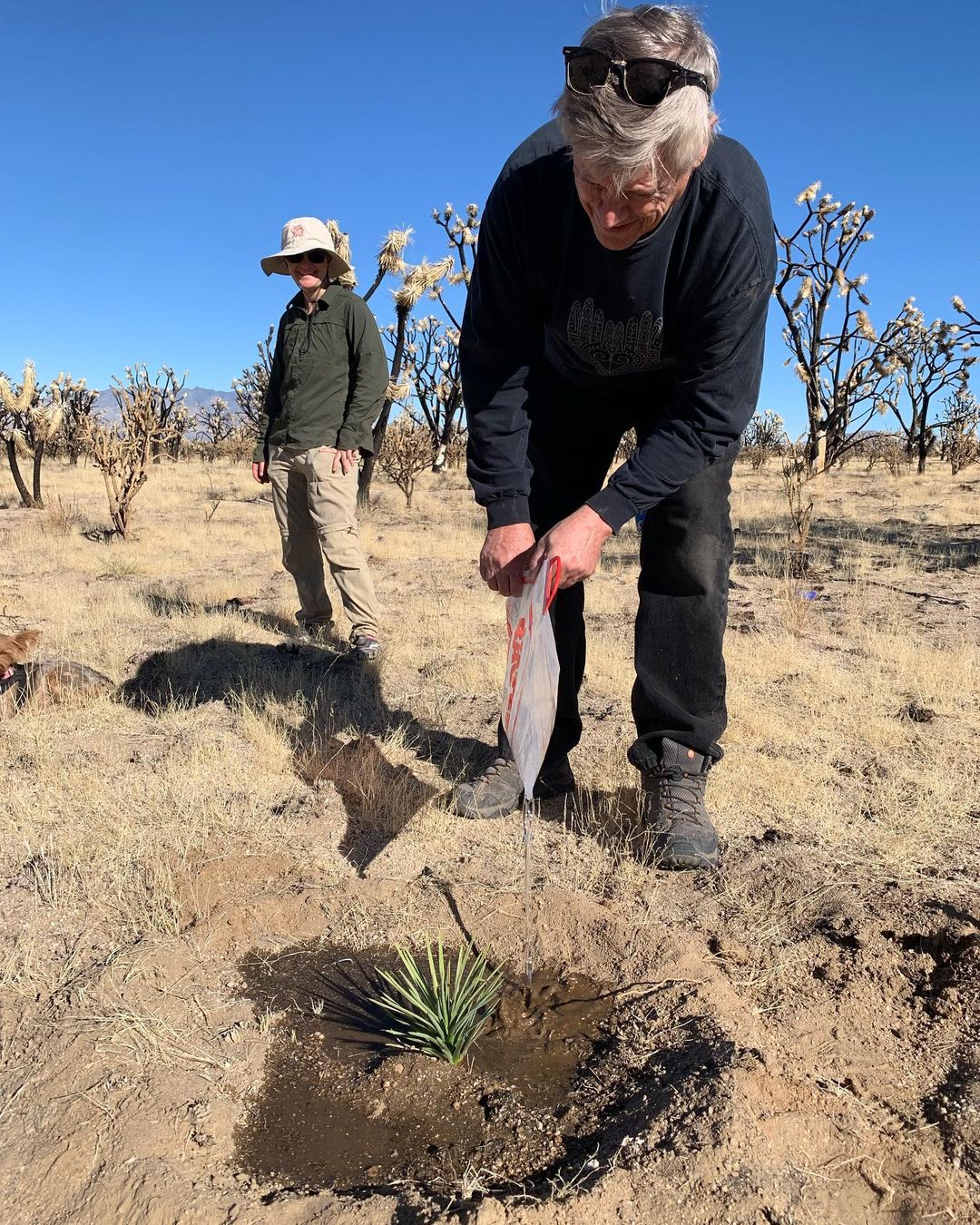In this desert photograph taken during either late winter or early spring, two older white men, appearing to be in their 60s, are the central focus. They stand against a backdrop of a brilliant blue sky and a ground that is predominantly dry and tan brown, laden with lifeless, dingy soil and sparse, dark, stemmy vegetation. The main point of interest is a small green shrubbery in the foreground, the only green amidst the arid landscape.

One man, dressed in black attire including a long-sleeve shirt, pants, and muddy boots, is slightly hunched over, tending to the shrub. He has gray hair, sunglasses resting atop his head, and appears to be watering the plant from a Ziploc bag, with the soil around the plant noticeably wet. The second man, standing behind him to the left, sports khaki pants, a dark green shirt or jacket, and a white canvas bucket hat. He is watching the first man with a smile, wearing his sunglasses and conveying a sense of support or camaraderie. The scene captures a moment of effort and care amidst a harsh environment, highlighting their endeavor to nurture life in the desert.